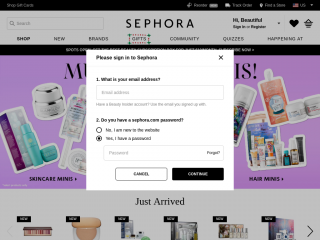This image captures a screenshot of the Sephora website. At the top, a prominent white banner stretches horizontally from left to right, featuring search options alongside tabs labeled "Shop," "New," "Brands," "Gifts," "Community," and "Quizzes." The main content area is partially obscured by a sign-in prompt asking users to enter their email address and password, with buttons to either cancel or continue the process.

In the blurred background, a variety of Sephora’s offerings are faintly visible, including categories like hair care, skin care, and minis. These items are presented in an assortment of sizes and colors, appearing somewhat jumbled together. Near the bottom of the image, there is a section labeled "Just Arrived," though the specific products are hard to discern due to the image's blurriness.

Overall, the screenshot gives an overview of Sephora’s dashboard, highlighting key website navigation elements and a customer login prompt.